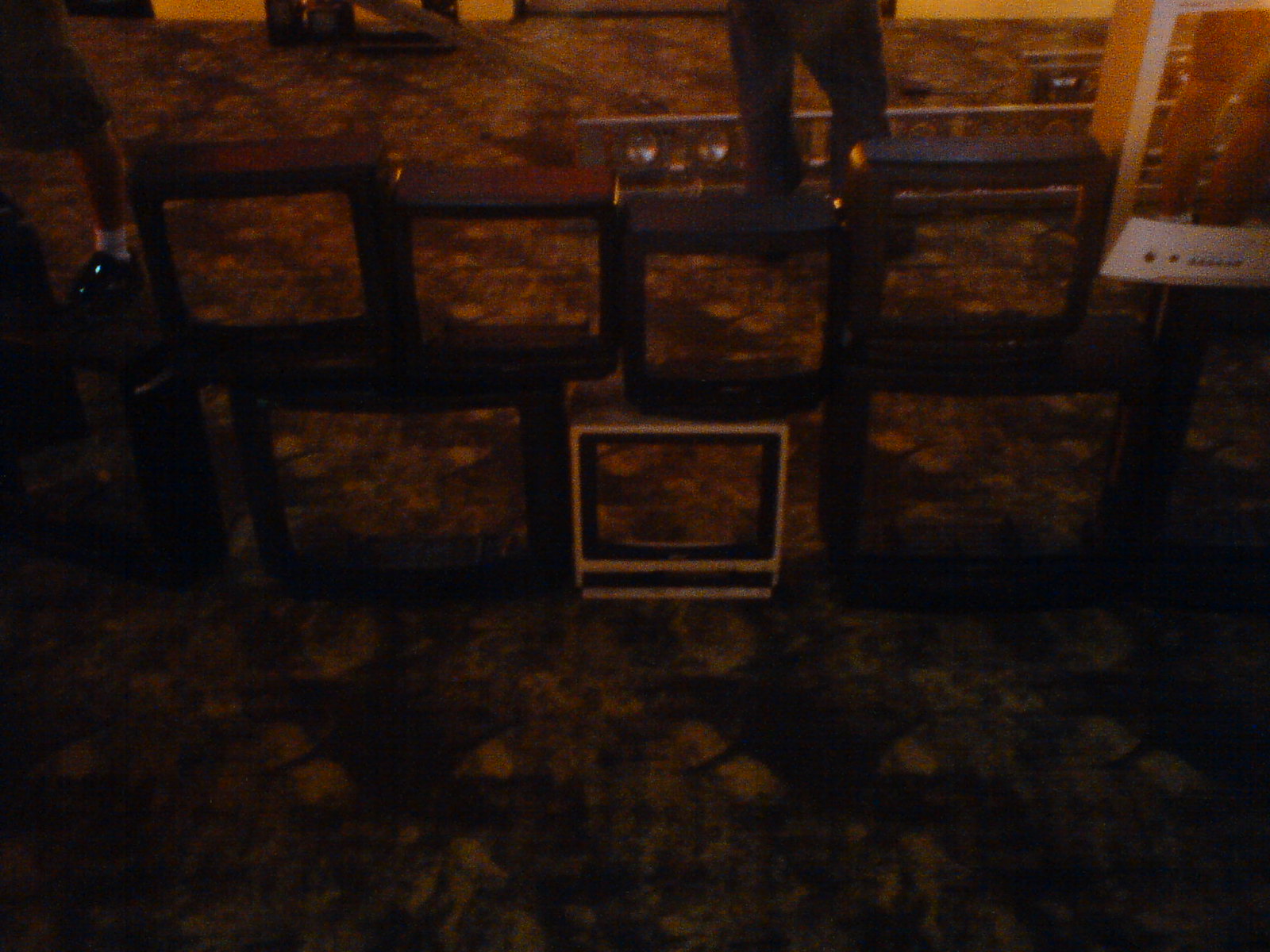The image depicts a dimly lit scene inside an antique store or possibly an electronics shop, where numerous vintage CRT TV housings, reminiscent of 1990s models and varying in sizes up to about 27 inches, are arranged in a conspicuous display. These seven or so CRT casings, stacked two-high and forming a modest tower, appear to be mostly hollow except for one which may still contain some internal components. The frames are predominantly black, except for a distinctive white-framed TV situated in the center of the bottom row. The background features a reddish-brown hue, suggestive of dry leaves scattered around, and a sleek steel light bar with a couple of spotlights aimed at the stack of TVs. Human legs are visible in the scene, indicating that someone is standing nearby, possibly inspecting this curious arrangement of nostalgic electronic artifacts.